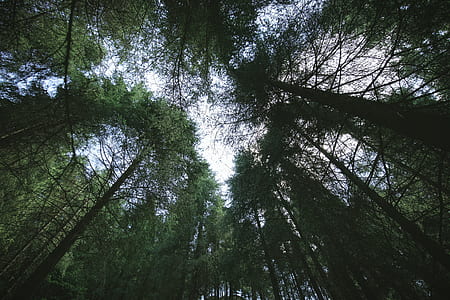The photograph captures a mesmerizing view from ground level, deep within a dense jungle. Taken during the day, the camera points upward, creating a circular or spiral perspective that draws the eye towards the sky, which appears white or faintly blue with some clouds. Surrounding the viewer, towering trees with almost black trunks and branches spread their dark green leaves into a canopy. The trunks are notably thin and the branches, some bearing leaves and some bare, fan out around the edges of the image. This intricate interplay of tall, slender tree trunks and lush foliage against a subtly clouded sky encapsulates the wilderness's raw and immersive beauty.